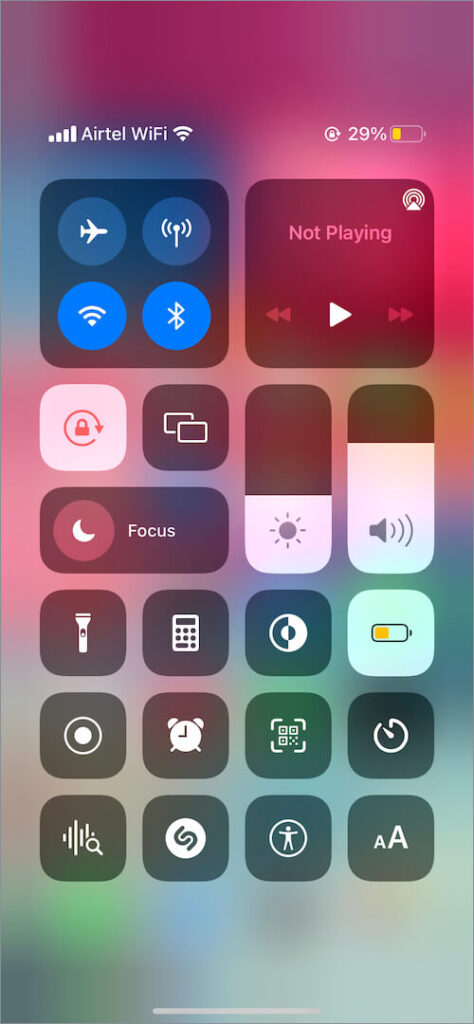The image features a screenshot from a cell phone, prominently displayed against a stark white background. The phone's wallpaper showcases a stunning abstract design, with soft, cloud-like transitions of colors — starting with muted pinks and purples at the top, blending into blue in the middle, and culminating in pinks and greens at the bottom.

In the top left corner of the screen, the status bar indicates four signal bars lit next to the word "Airtel." To the right, the Wi-Fi icon is fully lit, signaling strong connectivity. In the top right corner, a battery icon reveals a 29% charge remaining.

Just below the status bar, a rectangular black box presents four toggle options: "Airplane Mode," "Cellular," "Wi-Fi," and "Bluetooth." Each toggle is displayed clearly for easy access.

Adjacent to this panel, another black box appears with the text "Not Playing" in red, adjacent to a white play button. Beneath this, a smaller section displays several icons, including a prominent black box housing the letter "A" in white and a circular icon with a white-outlined human figure on the left.

Overall, the image intricately details the phone's interface against an ethereal and serene abstract background.